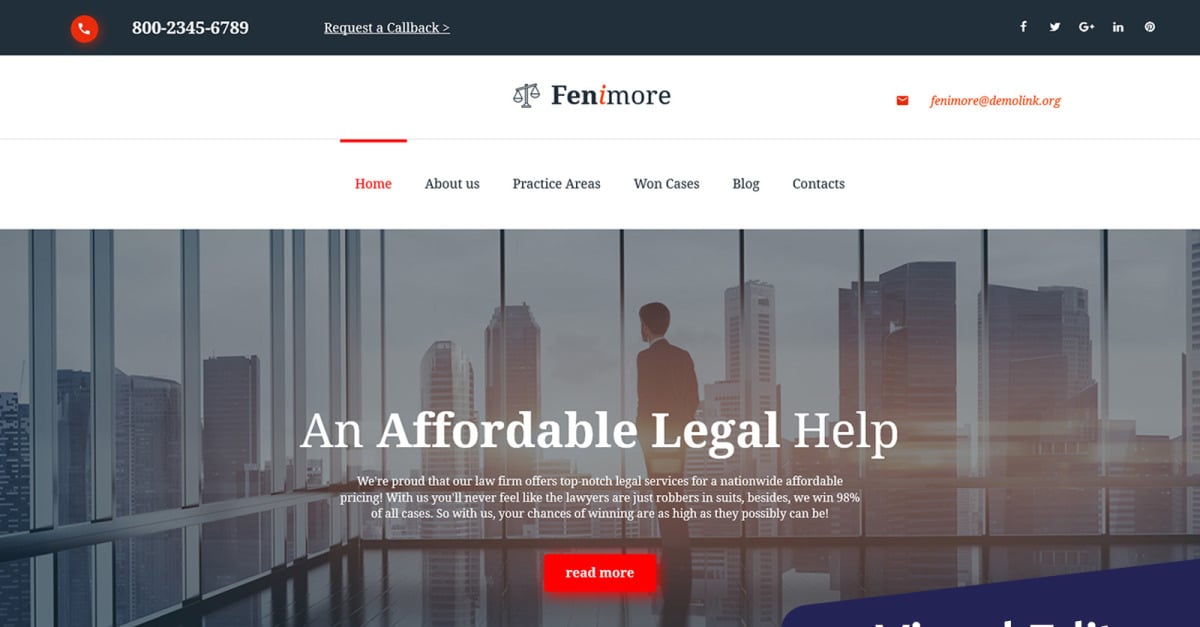The webpage features a prominently placed black banner at the top. Inside the banner, there's a small red circle with a white phone graphic and the text "800-234-56789" in white. To the right of this, the phrase "Request a callback" is underlined and accompanied by a right arrow. On the opposite side of the banner, icons for Facebook, Twitter, Google Plus, and LinkedIn are displayed.

Beneath the banner, the page transitions to a white background. Centrally placed, in bold text, the name "Fenimore" is displayed. The letters "F-E-N" are in a bolder print, the letter "I" is in red, and "more" appears in a thinner font style. 

On the right side, there is a red envelope icon with the email address "Fenimore@Demolink.org" written in orange text.

Further down, a horizontal line separates the sections. Directly beneath this line is a navigation menu with the options: Home, About Us, Practice Areas, One Class, One Cases, Blog, Contacts. 

The central image on the page shows a modern office building with a man gazing out the windows towards the city. Underneath this image, the text reads "An Affordable Legal Help" followed by a brief descriptive paragraph about the services offered. A red button with the text "Read More" in white invites users to explore further.